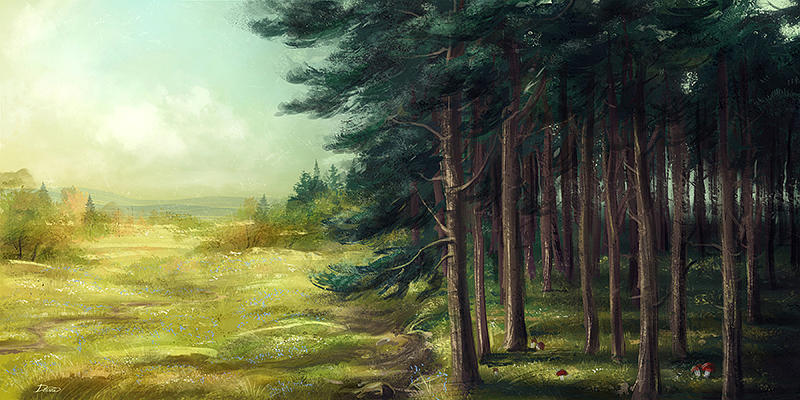This painting depicts a serene landscape split between a rolling meadow on the left and a dense forest on the right, encapsulated within a long, narrow horizontal rectangle. The meadow, vibrant with shades of light and medium olive green grass and speckled with sun-kissed patches of yellowish-green, stretches toward the background where clusters of small trees and a quaint cottage with a triangular roof are nestled. Gentle hills and bumps contour the land, giving it a lush, undulating texture. Above, the sky occupies the top left quadrant, painted with soft hues of pale blue and scattered with clouds.

Dominating the right half of the painting is a thick forest of towering evergreen trees, characterized by their straight, dark brown trunks and dense foliage clustered mostly at the top. The forest floor, a dark olive carpet of grass or moss, shifts in tone with the play of sunlight filtering through the canopy. Sunlight casts sharp shadows, adding depth and contrast, and dots of sky peek through the tall pines, especially in the distant right.

In the far background, a hint of distant mountains emerges, veiled partially by high clouds. The entire scene evokes a peaceful, idyllic natural setting, suggesting a valley that sits comfortably between two mountain chains, bathed in soft daylight. The forest appears tidy and traversable, inviting a leisurely walk under the sun.